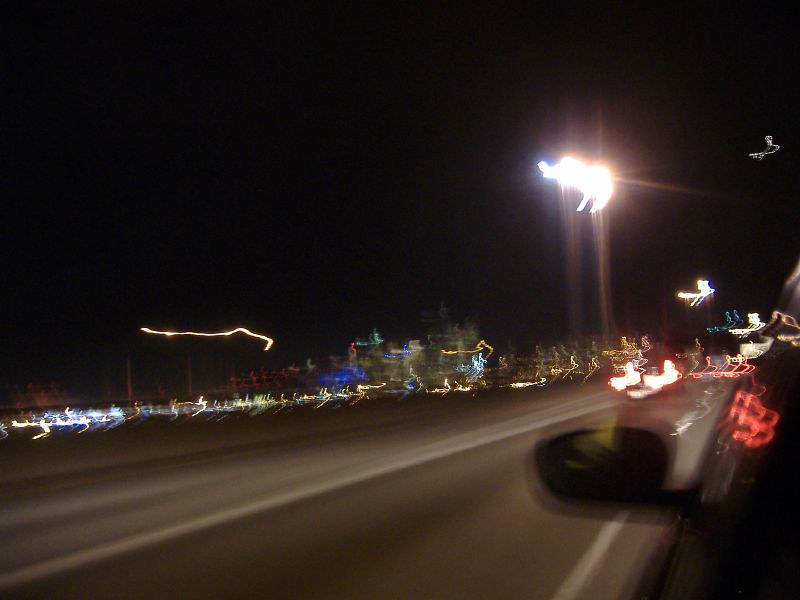This nighttime photograph, taken from a moving car, has an ethereal, blurred quality due to motion and possible digital effects. The dark black sky forms a backdrop to a scene filled with streaks of light. The lower right corner of the image shows the black exterior and side mirror of the car, with a glimpse of the dark gray asphalt road, marked by white lines, running alongside.

To the left, there's a series of trailing lights that include bright, wispy brake lights from a line of cars at what might be a stoplight transitioning to green. These lights extend into the background, mingling with blue, yellow, green, and white lights that could belong to cars or small buildings. This colorful array forms jagged, streaked lines, enhanced by the blur.

An outlined silhouette of trees appears dark green against the night sky, interspersed with blurry images of buildings. Bright street lights are seen without visible bases, and what might be a tall pole with two radiant lights crowns the top of the frame, casting rays that blend into the dreamy, unfocused composition.